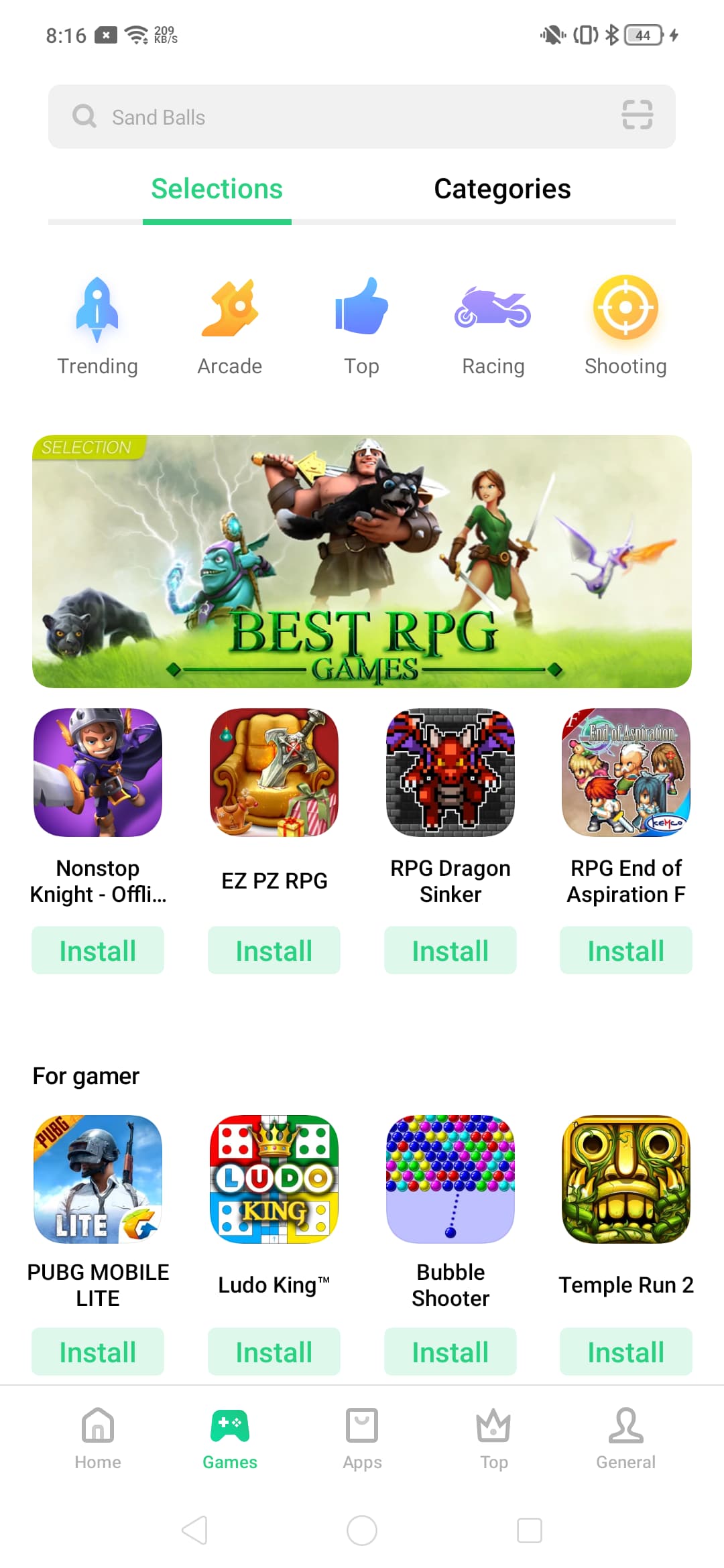**App Store Page Showcasing the Best RPG Games**

**Header Description:**
The app store page is dedicated to highlighting the best RPG games, featuring a lush green grass background. The header reads "Best RPG Games" in bold, green fonts. To enhance the design, horizontal green lines flank the word 'Games,' each terminating in a diamond shape, slightly extending beyond the text. A light, cloudy sky forms the background, punctuated by thin, subtle lightning bolts on the left. In the upper left corner, a small green box with the word "Selection" in white text is visible.

**Featured Characters:**
The page showcases five RPG characters against this ethereal backdrop:
1. A foreboding black tiger-like creature that exudes an eerie vibe.
2. A whimsical cartoonish goblin wizard with teal skin, wielding a staff that shoots out lightning bolts from its hands.
3. A classic, muscular warrior holding a black dog in his left hand, with an axe or similar weapon slung over his right shoulder.
4. A young, athletic female warrior brandishing two swords—one facing downward in her right hand and the other facing upward in her left.
5. A diminutive purple dragon spewing fire from its mouth.

**Navigation Bar:**
The top navigation bar displays standard cell phone information:
- Time: 8:16
- Icons: YouTube, Wi-Fi, 209 KB/S (possibly the internet speed), alarm (canceled), reorientation, Bluetooth, and battery status showing 44% with a power icon adjacent.

**Search and Tabs:**
Below the header, a search bar features a gray magnifying glass icon, with the text "sandballs" entered. Two tabs are available: 
- "Selections" (currently highlighted in green)
- "Categories."

**Action Buttons:**
A row of action buttons is present, each with an icon and label:
- Trending (blue rocket ship)
- Arcade (orange-yellow racing shoe)
- Top (blue thumbs up)
- Racing (purple motorcycle)
- Shooting (white bullseye inside an orange circle).

**Main App Display:**
Following the action buttons is the main image described earlier, followed by a neat 2x4 layout of various apps, each accompanied by a green "Install" button. The featured apps include:
- Non-Stop Knights: Offline, Easy Peasy
- RPG Dragons Sinker
- RPG End of Aspiration F

**For Gamers Row:**
Another row labeled "For Gamers" contains the following apps:
- PUBG Mobile Lite
- Ludo King
- Bubble Shooter
- Temple Run 2

**Bottom Navigation Bar:**
At the very bottom, a navigation bar includes:
- Home icon
- Games (highlighted in green with an Xbox-like controller icon)
- Apps
- Top (with a crown icon)
- General (featuring an outline of a person's shoulders and head)

**Media Controls:**
Beneath the bottom navigation bar, media control buttons—Play, Record, and Stop—are outlined in thin gray, filled with white.

This detailed layout delivers a rich and engaging user experience for RPG enthusiasts searching for their next adventure game.